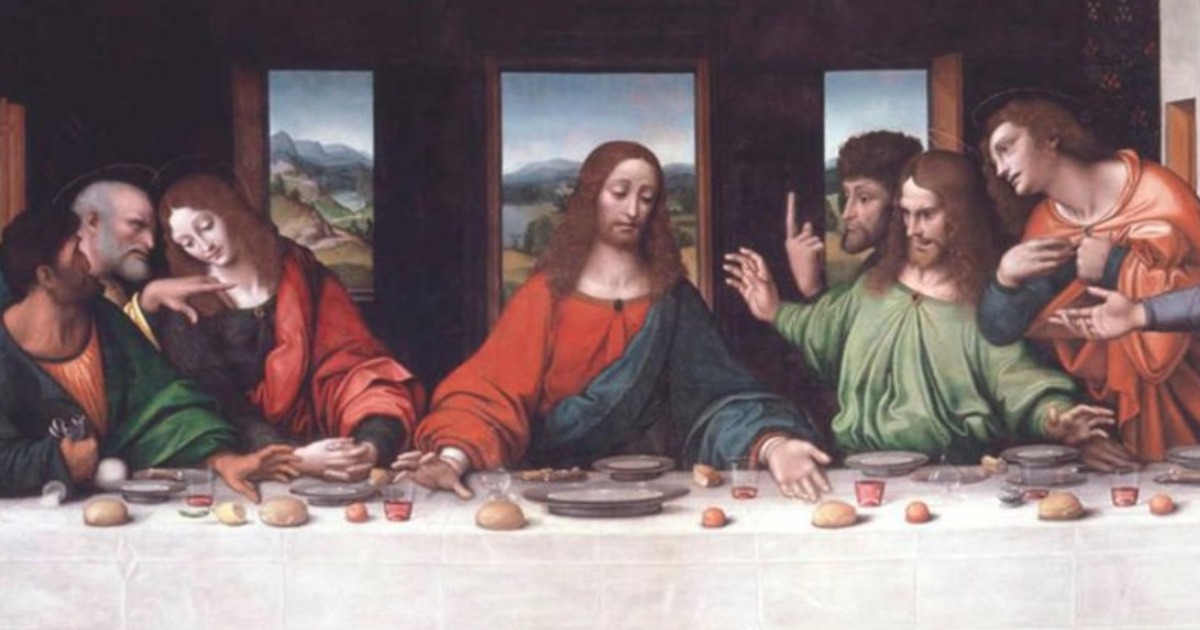This image is a detailed illustration of Leonardo da Vinci's "The Last Supper," capturing an ancient scene with incredible nuance. The rectangular painting portrays Jesus and his disciples gathered at a long table covered with a white cloth. The table is set with gray metal dishes, plates, and glasses filled with red liquid, likely wine, as well as scattered rolls of bread and potatoes. Jesus, the central figure, has long brown hair and wears a red flowing shirt with a blue toga draped over his right shoulder. On either side of Jesus, three disciples are engaged in conversation, leaning in and pointing towards him, emphasizing his role as the focal point. The disciple to Jesus' immediate right wears a green tunic and has long hair, while others are depicted in ancient robes with varied gestures and expressions. The background features dark walls with cutouts for windows, revealing picturesque nature scenes including mountain ranges, hills, and trees, enhancing the serene yet poignant atmosphere of the scene.